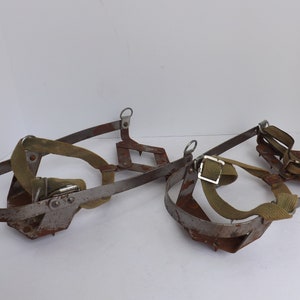The image depicts two identical metal contraptions lying side by side on the white floor of an empty room, with stark white walls adding to the minimalistic setting. The contraptions, which bear a resemblance to old leg braces or harnesses, are primarily composed of weathered, rusted metal, forming a roughly U-shaped structure where two metal pieces curve downward and meet at the bottom. Each contraption features green straps interwoven with the metal frame, possibly suggesting adjustable supports, and a leather strap with a buckle that might have been used for fastening. The objects are positioned horizontally across the base of the image, emphasizing their aged and utilitarian design amidst the clinical, unembellished backdrop.